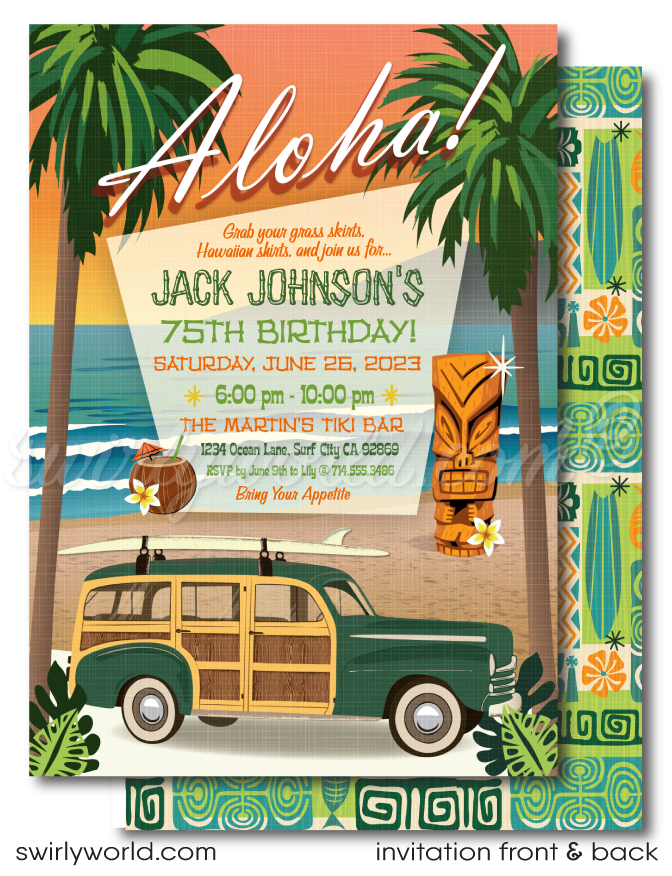This vibrant cartoon-style invitation, themed around a Hawaiian luau, invites guests to Jack Johnson's 75th birthday celebration. Featuring bold, colorful illustrations, the image showcases the word "Aloha" at the top, framed by an ocean sunset and waves. The central graphic includes two palm trees flanking a traditional tiki statue, with a coconut drink adorned with a straw and a flower beneath them. A classic green woody station wagon with wooden side panels sits at the bottom, adding a nostalgic touch. 

The invitation reads: "Grab your grass skirts and Hawaiian shirts and join us for Jack Johnson's 75th birthday, Saturday, June 25th, 2023, from 6 PM to 10 PM at The Mountains Tiki Bar, 1234 Ocean Lane, Surf City, California 92869. RSVP by June 9th to Lily at 714-555-3486. Bring your appetite."

The matching envelope is equally festive, decorated with bright green and orange geometric swirls, flowers, and surfboards. The back of the card and the invitation feature the website swirlyworld.com, merging vibrant designs with important event details.